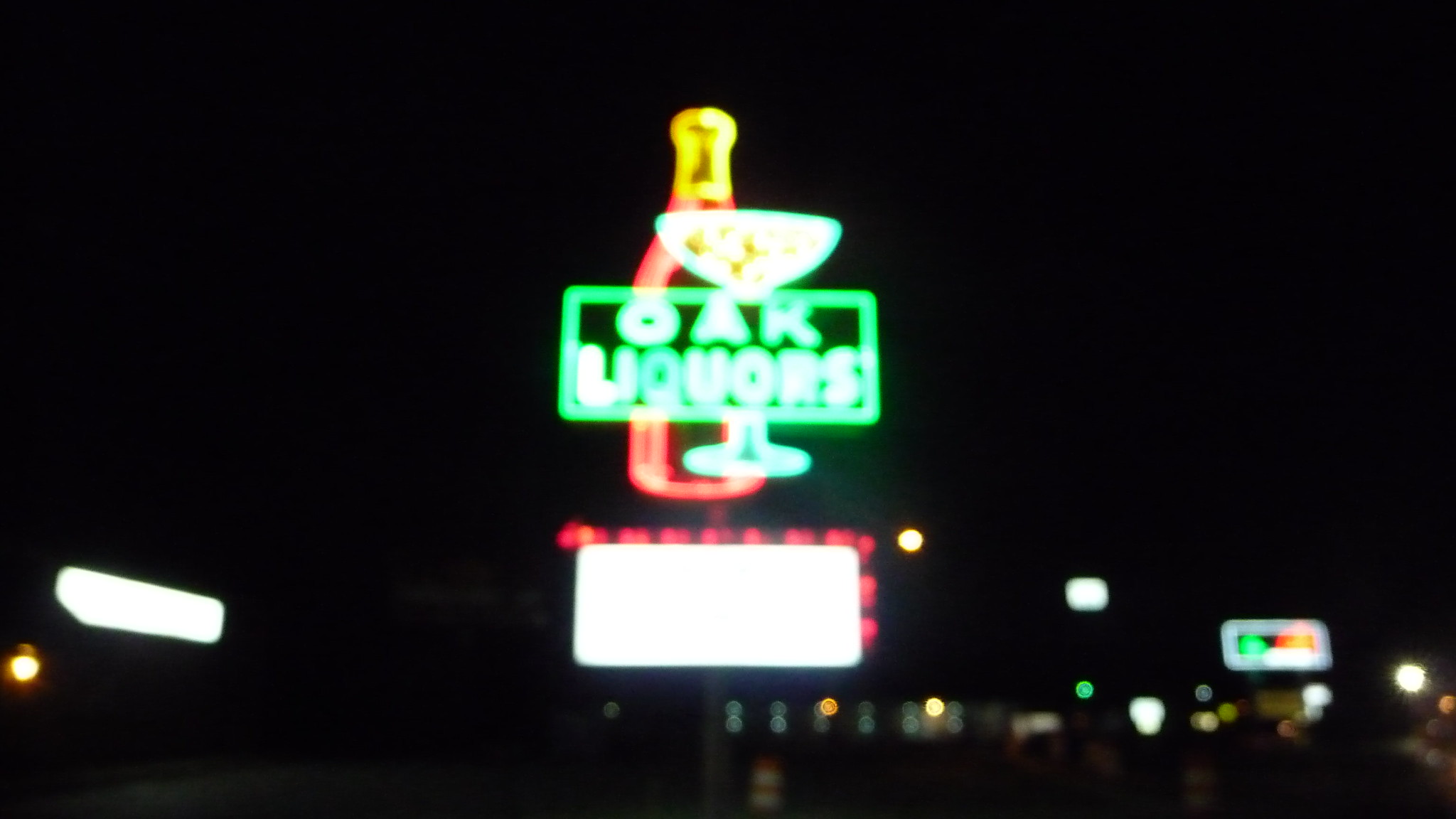A nighttime cityscape featuring a slightly blurry image of a neon store sign takes center stage. The imposing neon sign, mounted on a stand, is illuminated with vivid light green and light red colors. At its center, the sign prominently reads "Oak Liquors," underneath which an illustration of a martini glass and a champagne bottle glows, hinting at the store's offerings. Positioned directly below is a bright white rectangular sign, its content obscured and unreadable due to the bright illumination. The background reveals a mosaic of city lights from nearby buildings, with a long rectangular white light distinctly visible on the left, and a blend of various building illuminations scattered on the right. The dark, starless sky above adds a stark contrast, emphasizing the bright, lively atmosphere of the city at night.